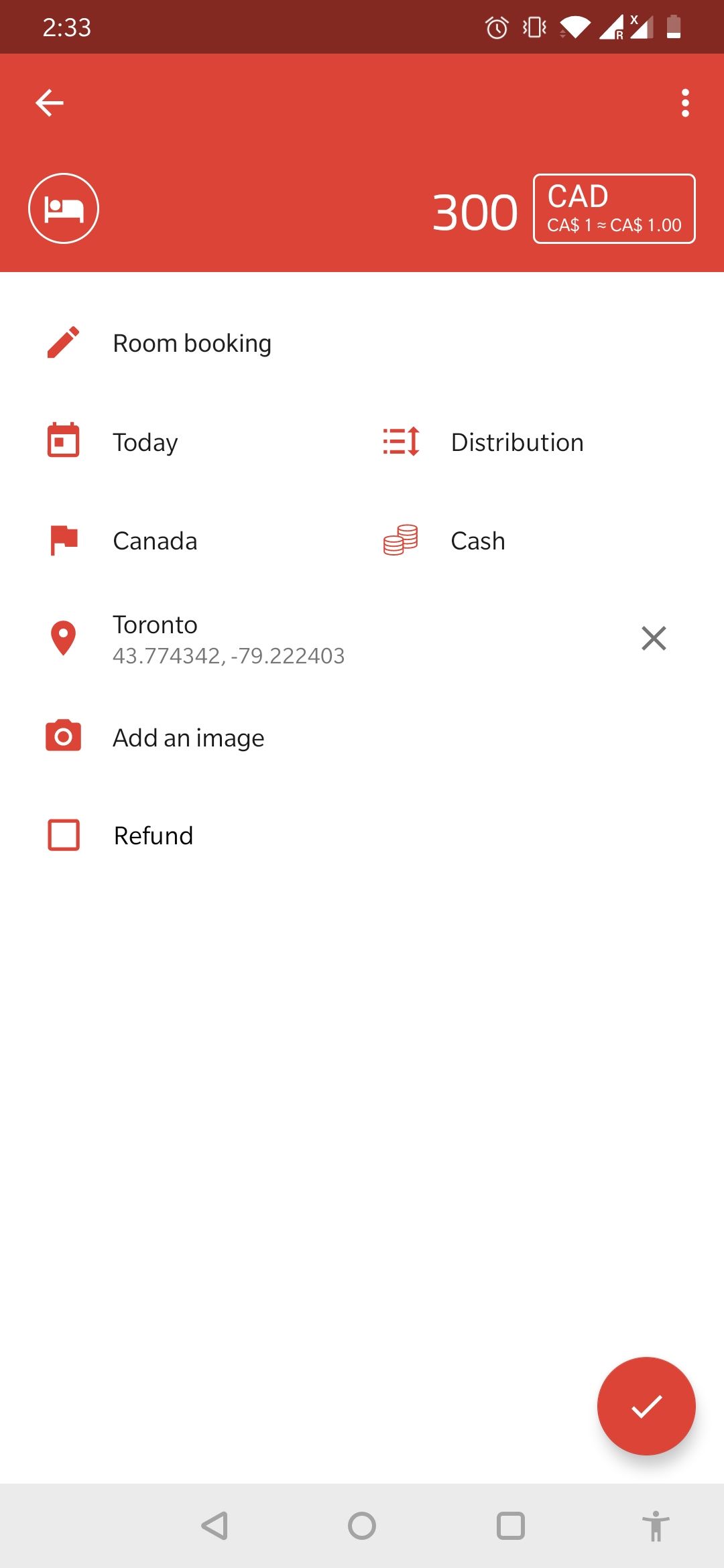The image is a screenshot from a smartphone displaying a webpage. The top header of the screen is a brick red color. The device's status bar at the very top shows the time as 2:33 on the left side, while the right side features various icons: a low battery icon (about one-quarter full, although the exact percentage isn't specified), wireless network and Wi-Fi icons, a mute icon indicating the phone is on silent mode, and an alarm clock icon.

Beneath the status bar, the website's header graphic also adopts a slightly lighter brick red hue. On the right side of this header, the text "300 CAD" (indicating Canadian dollars) is displayed in white font within an unfilled rectangular box.

Below the header, the main section of the webpage has a white background. The left side of this section lists several options in a gray font: "room," "booking," "Canada," "Toronto," "add an image," and "refund." On the right side, there are the words "distribution" and "cash."